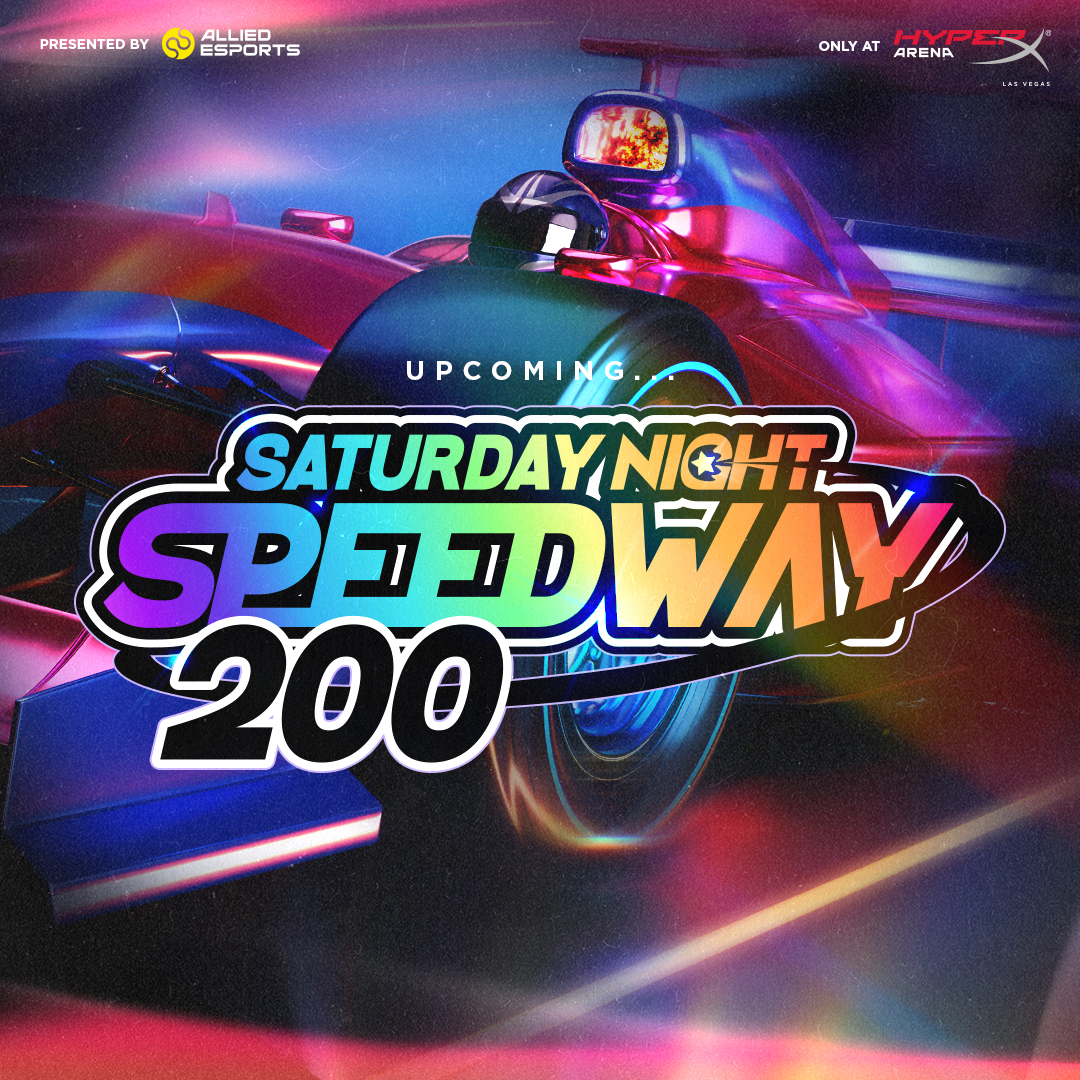This vibrant promotional graphic is an advertisement for a racing event titled "Saturday Night Speedway 200," presented by Allied Esports. The main text, "Saturday Night Speedway," stands out with its vibrant rainbow colors ranging from red to purple, while "200" is displayed in bold black text with a white outline, slightly overlapping the word "speed." In the top left corner, small white text states "Presented by Allied Esports," and the top right corner reads "Only at HyperX Arena Las Vegas," linking the event to its venue in Las Vegas. The background features a glossy, toy-like Formula 1 race car, predominantly pink with blue accents, creating an energetic and dynamic atmosphere through motion blurs and glowing highlights. The front left tire of the car is centered in the image, detailed with a blue stripe around its very wide circumference. The track beneath, depicted in black, has white lines to the right, adding to the racing theme. Overall, the image exudes excitement and energy, making it an enticing invitation to the upcoming event.